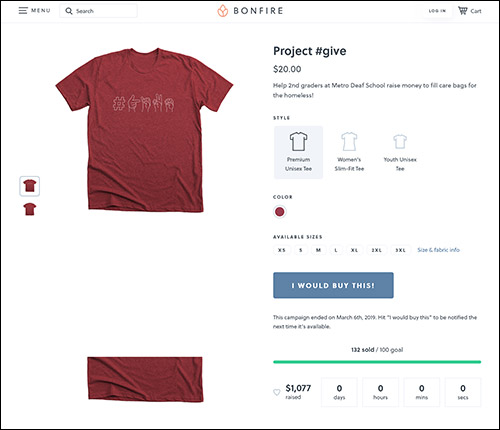The image showcases a slightly horizontally rectangular frame, appearing to be a screenshot from an item retail product listing page. In the upper left corner, the menu icon and search field are visible. Centrally, the Bonfire logo and "Bonfire" text are prominently displayed. The upper right corner features the login and cart options.

The main content of the frame focuses on a burgundy-colored t-shirt positioned on the left side. To its right, bold text reads "Project #Give," followed by a price tag of "$20." The description beneath this emphasizes a charitable cause: "Help second graders at Metro Deaf School raise money to fill care bags for the homeless."

Below this description, three t-shirt style options are presented side by side: "Premium Unisex Tee," "Women's Tee," and "Youth Unisex Tee." Although the color selection is limited to burgundy, a range of sizes is available: extra small, small, medium, large, extra-large, 2XL, and 3XL. A link for detailed size and fabric information is also provided.

At the bottom of the listing, a prominent blue button reads, "I would buy this."